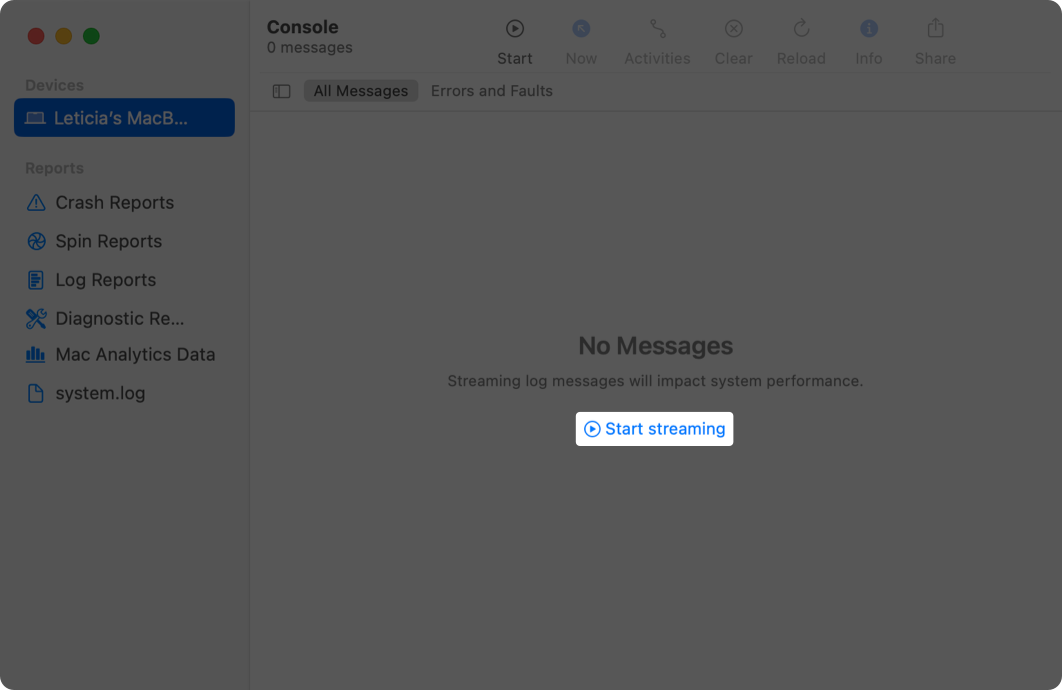In this screenshot, we see a user interface that appears to be a diagnostic or monitoring tool on a MacBook. At the center of the screen, there is a prominent blue button labeled "Start Streaming" with a play icon next to it. The surrounding area is grayed out, implying that the user must click "Start Streaming" to initiate any further actions.

In the upper left corner, there are three dots—red, yellow, and green—indicating that this is likely a screenshot from a MacBook. Below these dots, we see a sidebar categorized into sections starting with "Devices," where "Letitia's MacBook" is currently selected. 

Following that, there are various report categories listed under "Reports": 
- "Crash Reports" marked with a warning sign,
- "Spin Reports" symbolized with a spinning fan icon,
- "Log Reports" represented by bars on a piece of paper,
- "Diagnostics and Re..." with an icon showing a screwdriver and a wrench,
- "Mac Analytics Data" indicated by a bar graph,
- "System Log" shown with a piece of paper icon.

At the top of the screen, a menu bar features options from left to right: "Start," "Now," "Activities," "Clear," "Reload," "Info," and "Share."

Below this menu, the primary section is labeled "All Messages," which is currently selected, and adjacent options include "Errors" and "Faults." A message at the bottom states, "No messages. Streaming login messages will impact system performance," suggesting that initiating the streaming function may affect system performance. This screenshot provides a detailed view of the interface, likely intended for system diagnostics or log monitoring, rather than sharing text messages.